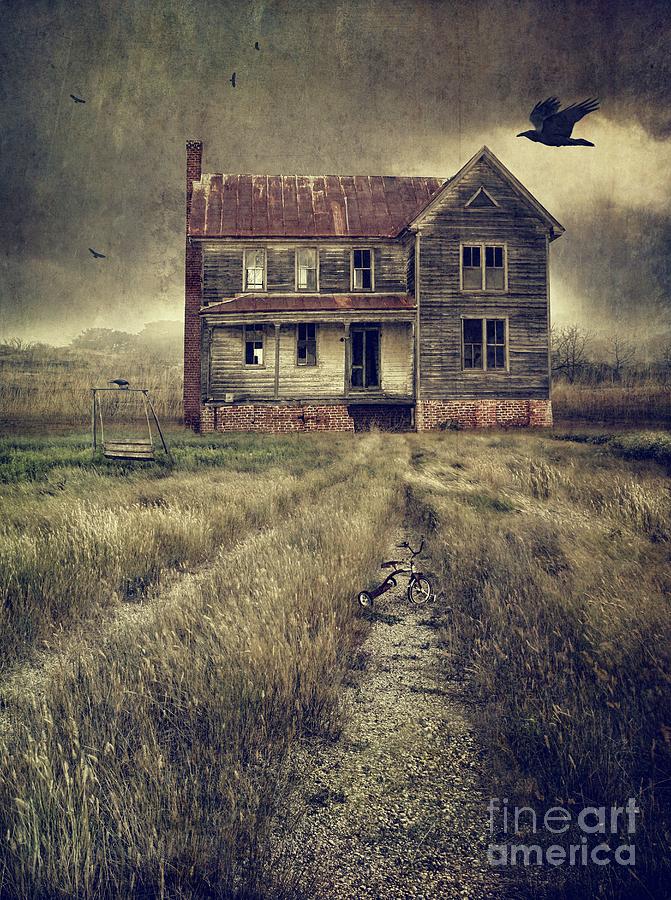The vertical rectangular image depicts a very old, abandoned wooden house with a brick foundation, rendered in sepia tones. The reddish roof has lost many of its shingles, and a tall chimney extends from the ground up the left side of the structure. The house, which misses many window panes, stands amidst overgrown weeds and an unharvested field, accessible via a gravel path. In the foreground, a tricycle rests on the pathway. To the left, a rickety, abandoned swing set, with a crow perched on it, adds to the eerie atmosphere. Several crows fly above the house against a dark, cloudy gray sky. The image bears a watermark in white semi-transparent letters that reads "Fine Art America" in the bottom right corner. The photograph seems digitally enhanced to give it an old film style, complete with lines across the screen, augmenting the haunted aesthetic.